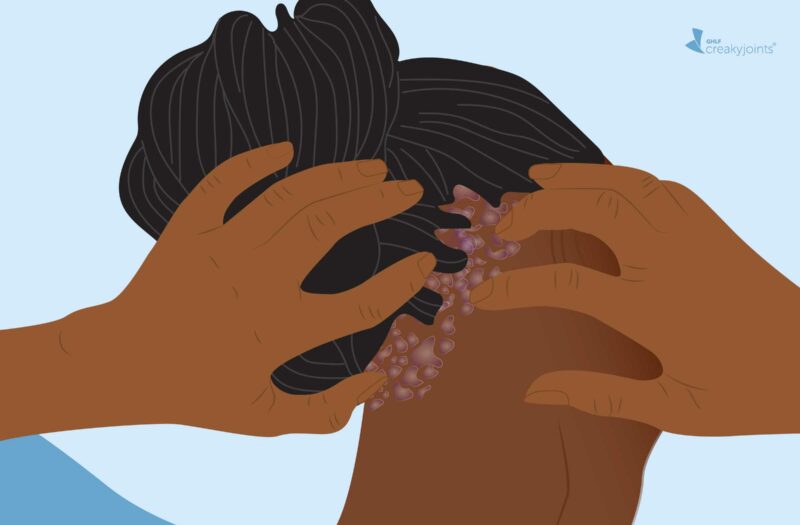The digital illustration depicts the back of a dark-skinned person washing their long black hair, which is wrapped up into a bun. The person is using their hands to massage purple, bubbly shampoo into the base of their hair, with numerous bubbles visible along the back hairline. One hand is holding up the hair while the other scrubs at the scalp, revealing several red bumps or polyps along the edge of the hairline. The background is a bright sky blue with a darker blue corner on the bottom left. Text in the top right corner reads "GHLF Creaky Joints" accompanied by a small blue abstract logo beside it. The person's face is not visible, only their neck, hands, and the back of their head and scalp.